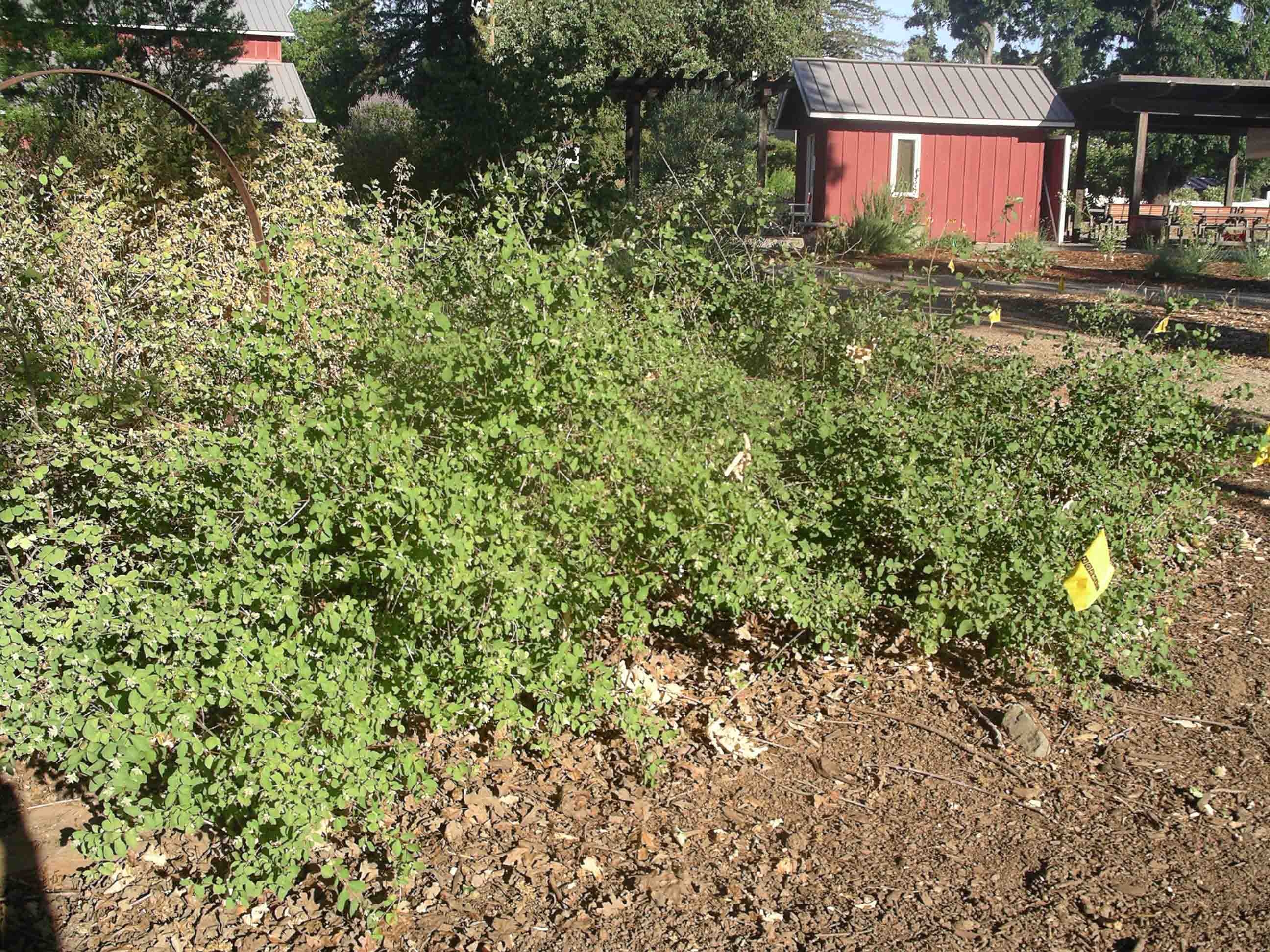The image captures a tranquil, rustic outdoor country setting. In the foreground, a small hillside is densely covered with vibrant green vegetation, punctuated with some small flowers. To the left, tall green weeds and small leafed plants grow robustly from a medium brown dirt patch that includes scattered leaves and a rusted circular object, reminiscent of a giant wheel frame. A dirt path runs from the left of a red shed with wood paneling and a gray, triangular roof, extending beyond the right edge of the image. Adjacent to the shed is a covered outdoor seating area. In the background, partially obscured by thick shrubberies and tall trees, there's a larger red building, likely the main farmhouse, with a light gray roof. The clear blue sky peeks through the upper part of the image, completing the serene scene. In the bottom right corner of the photo, a small yellow tag lies atop the greenery, its purpose unclear.